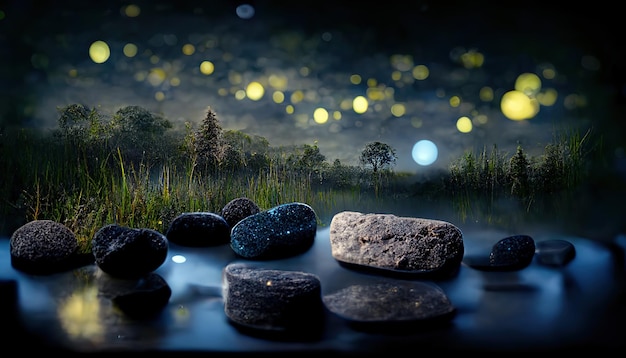The image appears to be an AI-generated night scene, characterized by an almost surreal blend of elements. In the foreground, there are numerous small, colorful stones resting on a smooth, glossy surface that might be water, suggesting a still or frozen appearance despite the absence of cold or snow. Among these stones, the largest one, centrally positioned, exhibits a mix of brown and dark brown hues, while a large, sparkly black stone is situated to its left. Flanking these are smaller stones, including a flat coin-like one and several others scattered around.

The background transitions into overgrown greenery with tall grass and trees, creating a dense, forest-like middle ground. Amidst the trees, a body of water might be faintly visible. Dominating the upper portion of the image is a night sky filled with semi-transparent, golden-yellow and light gray orbs that mimic stars or possibly glow bugs, adding to the otherworldly feel. The sky itself is a blend of blacks, navies, and blues, further distorted by the out-of-focus depiction of these orbs. Significantly, a white orb, presumably the moon, with an unusual bluish glow, hovers slightly to the right of center, enhancing the ethereal, somewhat off-kilter ambiance of the scene.